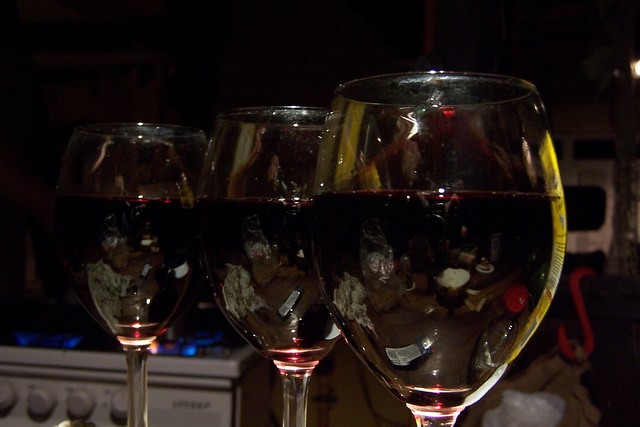The image depicts a close-up view of three transparent wine glasses, positioned side by side, each filled slightly more than halfway with what appears to be red wine. The glasses, with a fuller body that tapers at the top, beautifully reflect their surroundings within the liquid. The setting seems to be inside a bar, highlighted by the presence of a stereo or similar equipment with knobs and notable blue lighting in the background. The background itself is dark, emphasizing the clarity and reflective quality of the glasses, making them stand out. Despite some of the wine glasses partially obscuring their stems, the distinct reflections within the wine make for a striking visual, hinting at objects and perhaps a table beneath.